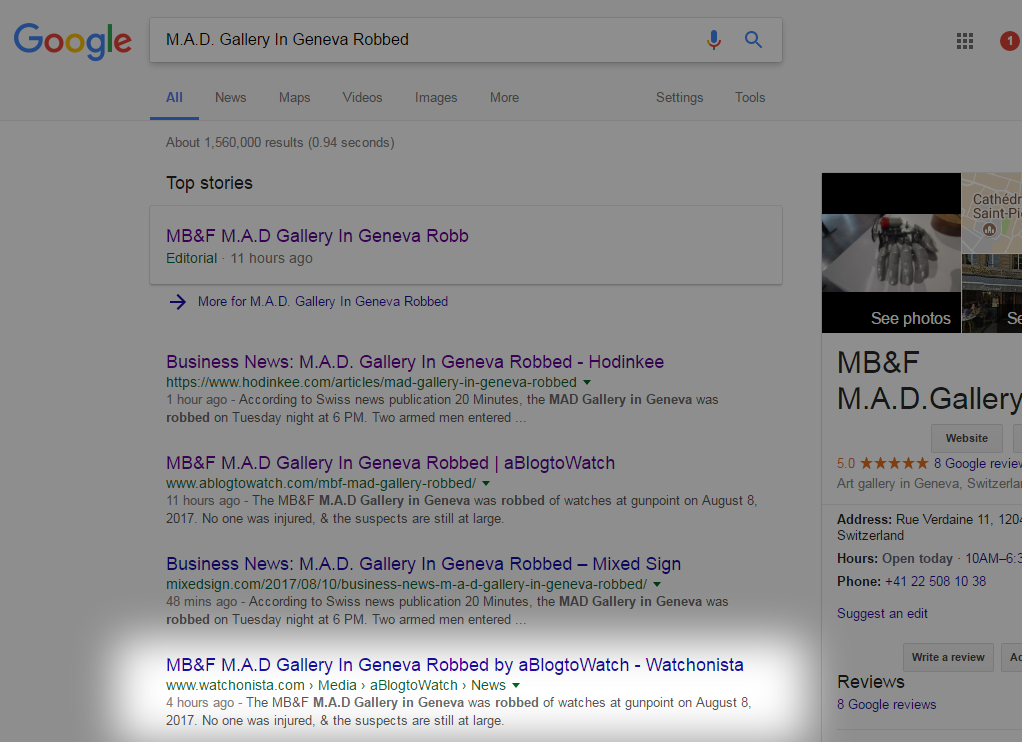**Screenshot of Google Search Results on the "MAD Gallery in Geneva Robbed"**

This image captures a partial screenshot of a Google search results page. The top-left corner prominently displays the iconic Google logo in primary colors, immediately identifiable alongside the search box containing the query "MAD Gallery in Geneva robbed." Adjacent to the search box are the microphone and magnifying glass icons. To the left, a few Google account-related symbols are visible, though specific account information is omitted.

Below the search bar, the following tabs are arrayed: All, News, Maps, Videos, Images, More, Settings, and Tools, with "All" currently selected. Beneath these tabs, it specifies that the search yielded approximately 1,560,000 results in 0.94 seconds.

The first result area is labeled "Top stories," highlighting a headline: "MB&F MAD Gallery in Geneva robbed - editorial, 11 hours ago," accompanied by a right-facing arrow indicating the option for "More for MAD Gallery in Geneva robbed." Following this, additional sources provide further information:

1. **Business News** - "MAD Gallery in Geneva robbed" by Honky D. Published one hour ago, citing Swiss News Publication, 20 Minutes, which describes an armed robbery at 6 p.m.
2. **A Blog to Watch** - "MB&F MAD Gallery in Geneva robbed," posted 11 hours ago, detailing the robbery of watches at gunpoint on August 8, 2017, with no injuries.
3. **Business News** - "MAD Gallery in Geneva robbed" by Next Sign, published 48 minutes ago, matching earlier details but mentioning suspects' arrests.
4. **Watchianista** - "MB&F MAD Gallery in Geneva robbed" again provides a highlight from A Blog to Watch, four hours ago, elaborating on the robbery's specifics and the current status of the suspects.

This particular result is accentuated with a bright white highlight, contrasting the otherwise muted, gray-shaded background.

To the right side of the screenshot, business information for the MB&F MAD Gallery is displayed, including options to "See photos," view the location on a map, visit the official website, and check out eight Google reviews averaging a perfect 5.0 stars. Additional details enumerate the gallery's address, operational hours, and contact phone number.

This meticulously detailed glimpse into Google's search result page serves as a comprehensive view of the widely reported robbery incident at Geneva's MAD Gallery.